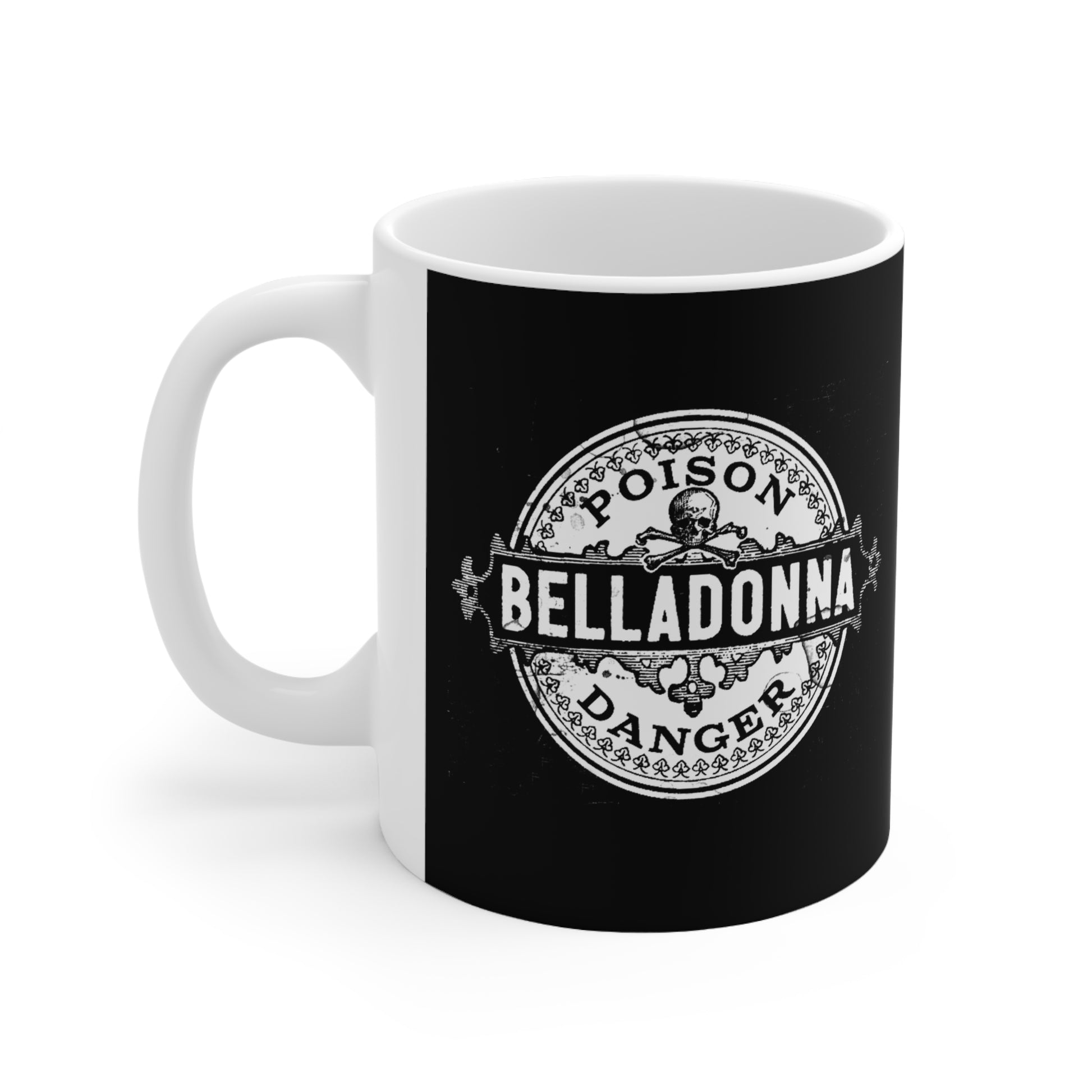This image features a striking black and white coffee mug placed against a white background. The ceramic mug predominantly appears in white, including the handle and interior, which are positioned to the left in the image. The most eye-catching detail is on the front section of the mug, which is adorned with a vintage-style design. This design includes a black rectangle serving as a backdrop for a white circular emblem. 

Prominently displayed within the emblem are the words "Poison" at the top and "Danger" at the bottom, each following the curved shape of the circle. A bold black band bisects the circle horizontally, bearing the word "Belladonna" in white lettering. Just above the band and nestled between the text "Poison" and "Belladonna," there is a detailed skull and crossbones illustration. Surrounding the inner circle, intricate filigree and leaf-like patterns add a touch of embellishment, reinforcing the design's old-school, vintage aesthetic.